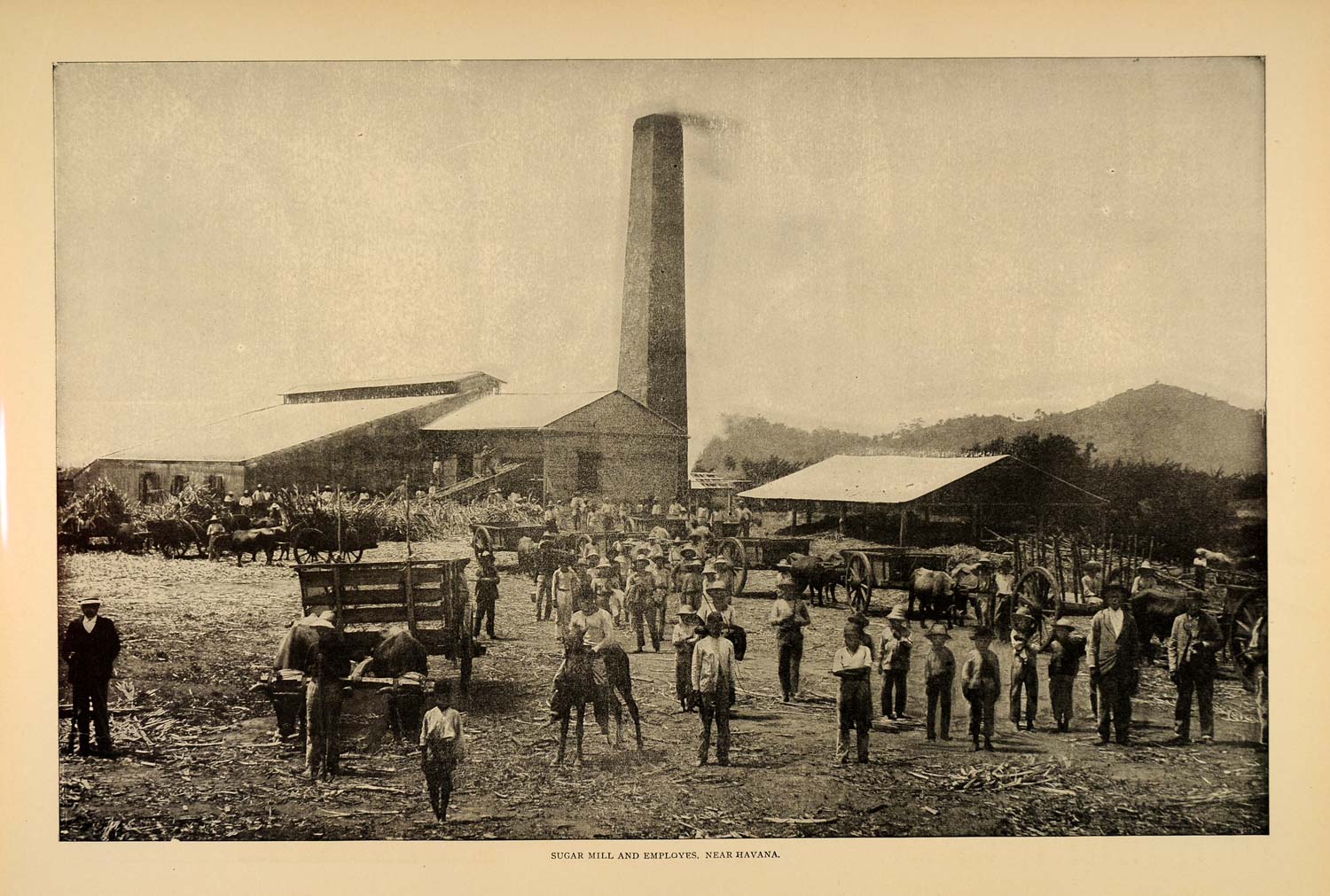This sepia-toned black and white photograph, which appears very old, depicts a bustling scene at a sugar mill near Havana. Dominating the background is a large building with a tall chimney emitting black smoke, accompanied by a ramp with people on it and numerous individuals milling around the premises. To the right, a farm is noticeable, and behind the activity, distant mountains frame the scene. Scattered across the foreground are about fifty men, mostly in their 30s or 40s, some possibly carrying guns. They are generally facing the camera but are not engaged in any specific activity. Among them and to the left are a few horse-drawn carts and wooden carriages. Animals, possibly cows or horses, are visible in the distance. The photo is labeled "Sugar Mill and Employees near Havana" at the bottom edge, capturing a vivid snapshot of agricultural and industrial life from a bygone era.